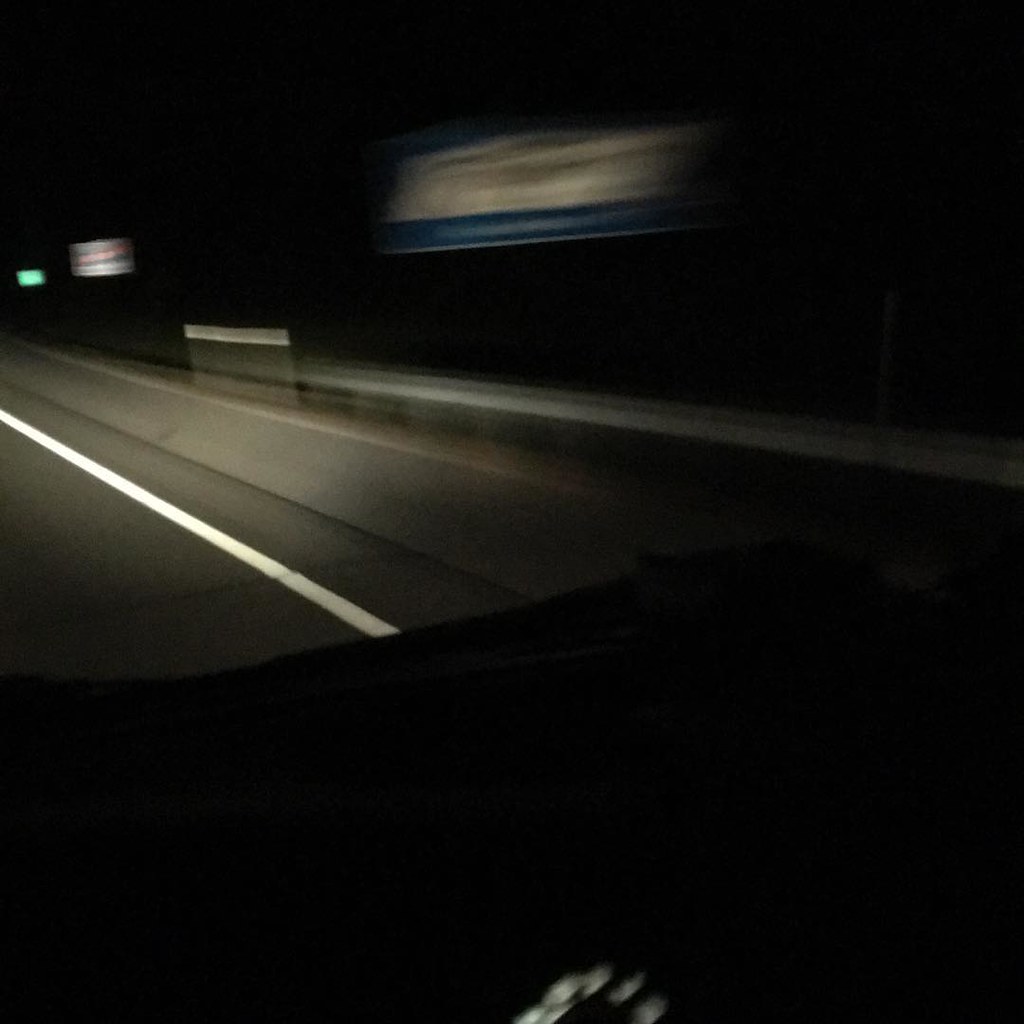A blurred nighttime photograph taken from inside a moving car, capturing the roadway ahead through the windshield. The interior of the car is shrouded in darkness, with indiscernible details except for a few white dots at the bottom, possibly indicating the speedometer. The car's headlights cast a light onto the gray paved road, revealing a white line running alongside. In the distance, the faint outlines of a gray guardrail and three signs — a blue and white one, a black and red one, and a green one — are visible, slightly distorted due to the motion blur.